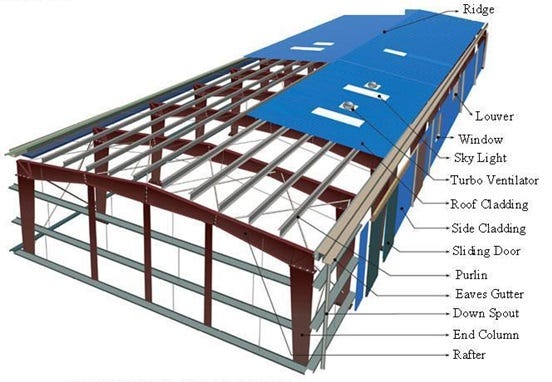This detailed architectural diagram showcases a comprehensive building structure rendered in shades of silver, burgundy brown, blue, and white. The image labels numerous parts of the building, with annotations in black font aligned from top to bottom, each connected by precise black lines. The components identified are: ridge, louver, window, skylight, turbo ventilator, roof cladding, side cladding, sliding door, purlin, eaves gutter, downspout, end column, and rafter. Despite a slightly grainy texture, the image quality remains crisp and clear, ensuring that all elements are distinctly visible and impeccably labeled.